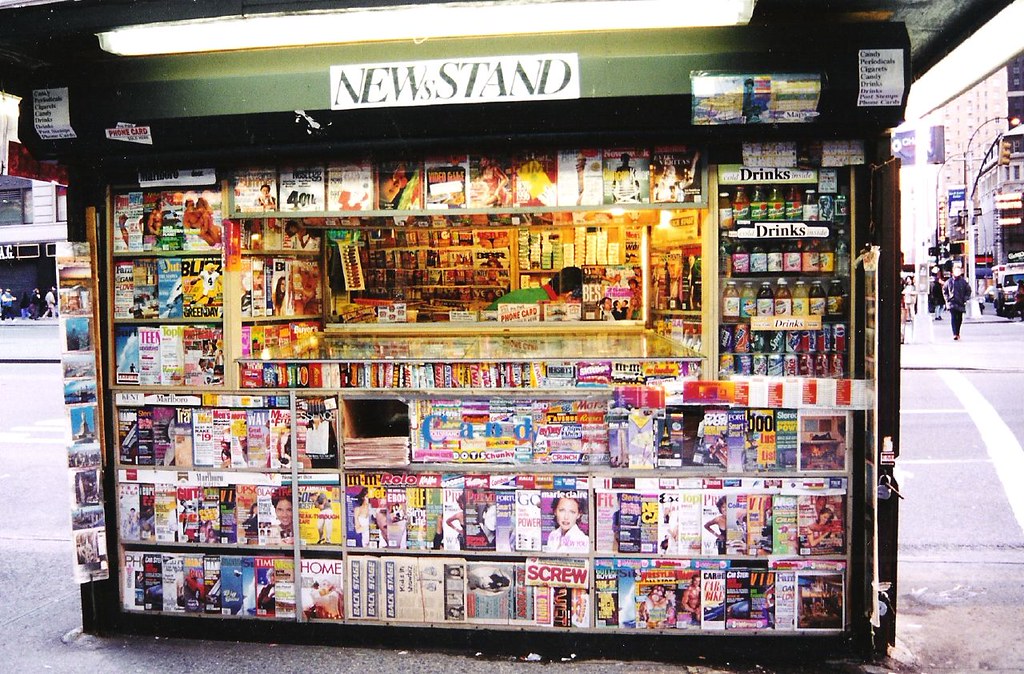This is a photo taken outdoors, depicting an urban city scene, likely from around 20 years ago or possibly longer, giving it an older feel. The focal point of the image is a green newsstand, labeled "Newsstand" at the top, situated on a city sidewalk with pavement visible on either side and a crosswalk to the right, suggesting it is at a corner. The background reveals some buildings, a road, and individuals standing on the sidewalk.

The newsstand is densely packed with numerous colorful magazines on display. Some recognizable titles include Time, Marie Claire, Teen Magazine, and Screw Magazine, indicating a possible 90s era as Teen Magazine has not been around for some time. In the center of the newsstand, there is a small window through which we can see part of a man with brown hair crouched down, possibly arranging items.

Apart from magazines, the newsstand also sells a variety of drinks such as Gatorade, Pepsi, Sprite, and Snapple. The right side has two labels with black text that simply read "Drinks." Additionally, candy bars are available for purchase. The top of the newsstand has some stickers, although their details aren't clear.